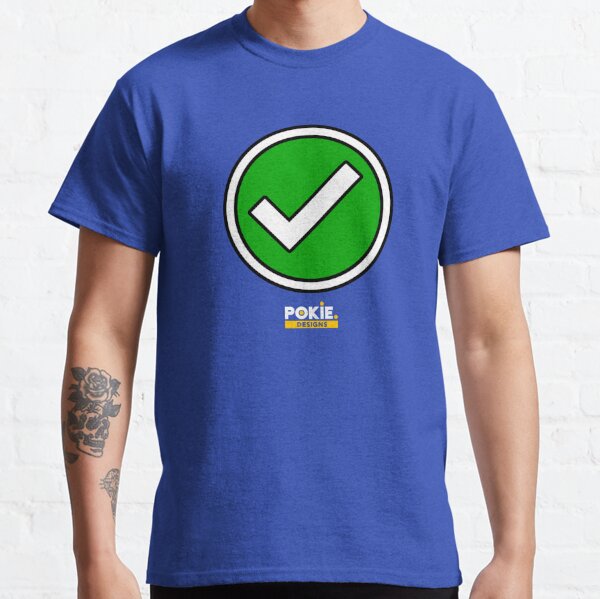The image depicts a man standing against a plain, stone-white background. He is wearing a blue t-shirt featuring a green circular emblem with a white check mark in the center, outlined in black. Below the emblem, the words "Pokie Designs" are written, with "Pokie" in a stylized font and "Designs" appearing on a yellow strip. On the man's right arm, there is a detailed tattoo of a rose with dark leaves and petals, set above a skull. There is also an additional tattoo below the main design, though its details are not clearly visible.